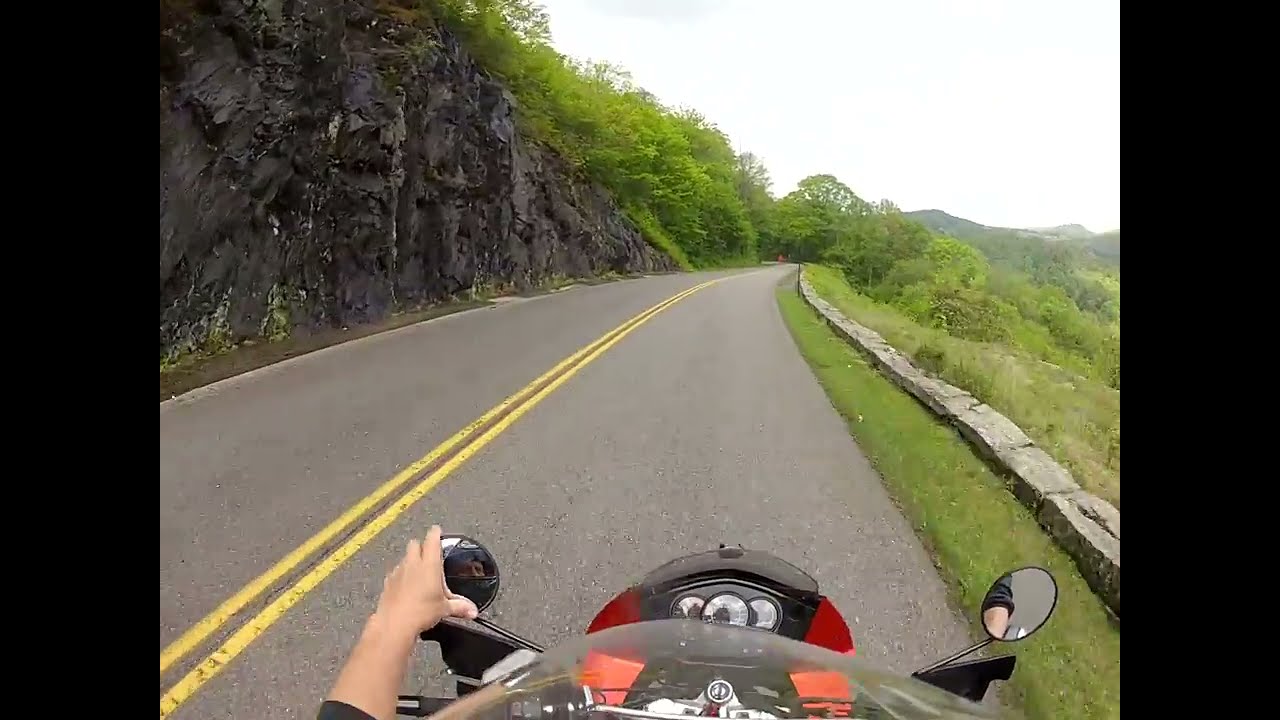The image is a first-person view from a driver riding a modern red and black sports motorcycle on a curved road. The driver’s left hand is visible, adjusting the left mirror, while the right mirror, handlebars, dashboard controls, and windshield are also seen at the bottom of the frame. The road is lined with two yellow lines, curving to the right. On the right side, there's a cliff with a brick or black wall, and a green field with short stones serving as a barrier. The left side of the road features a hard rocky cliff with bushes and greenery. The background showcases a clear sky, hinting at a remote mountainous area with abundant trees and overgrown grass, adding a sense of adventure and natural beauty to the scene.